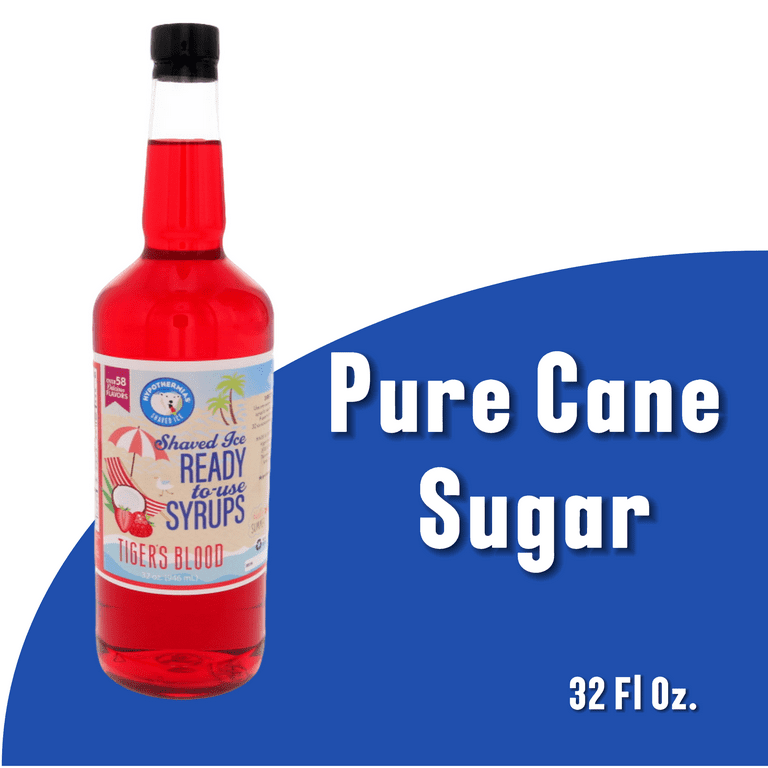This retro-themed advertisement showcases a glass bottle of "Tiger's Blood" ready-to-use syrup for shaved ice. The bottle, filled with a vibrant red syrup, features a black cap and an inviting beach-themed label. The label vividly depicts two palm trees, a beach umbrella with a towel, a beach chair, a seagull flying over sand, a coconut split in half, and two sliced strawberries, emphasizing the product's tropical fruit flavors. "Tiger's Blood" is prominently displayed in bold red letters on an oceanic backdrop. The ad itself is split between a blue background on the left and a white background on the right, with large white block lettering that proudly declares "Pure Cane Sugar," followed by the volume specification of "32 Fluid Ounces." The overall design exudes a nostalgic charm, reminiscent of the 70s and 80s era, making the syrup appear not only deliciously sweet but also nostalgically appealing.